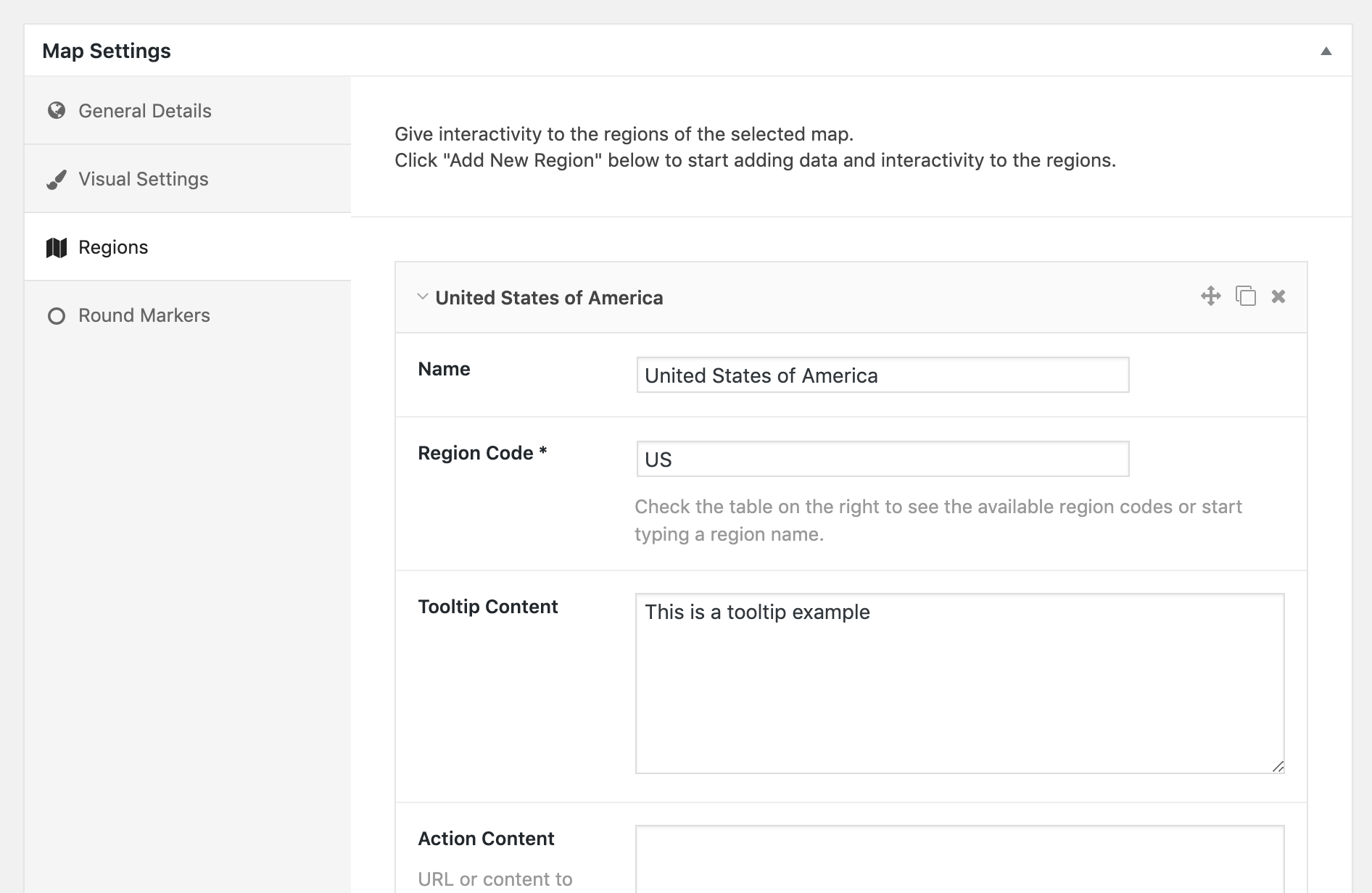The interface features a structured layout, predominantly outlined in light gray. At the top of the interface, a white rectangle titled "Map Settings" is positioned on the left side, accompanied by an upward-pointing triangle on the right side. Directly beneath this is a light gray rectangle labeled "General Details," which is indicated by an icon resembling a globe. Further down, another gray box marked "Visual Settings" is identifiable by an accompanying paintbrush icon.

Continuing downward, there is a white rectangle labeled "Regions," featuring what appears to be a wavy design. Below this is a long gray box with a darker gray-outlined circle labeled "Round Markers." As you shift your focus to the right, there is a larger white rectangle adjacent to two smaller gray rectangles. This larger rectangle contains the text, "Give Internationally to Regions of the Selected Map. Click 'Add New Region' below to start adding data interactively to the regions."

Further down, a light gray box with an arrow pointing downward is labeled "United States of America." To the left of this box are icons: a plus sign, two overlapping pieces of paper, and an X. Below these icons is a white rectangle titled "Name," followed by a smaller gray-outlined rectangle with the text "United States of America" inside it. An adjacent section reads "Region Code" with an asterisk, along with another small gray-outlined rectangle labeled "U.S."

Users are advised to "Check the table on the right to see the available region codes or start typing region names." Beneath this, under "Tooltip Content," is a larger rectangle outlined in gray with the example text "This is Tooltip Example." At the bottom of the interface, the section marked "Action Content" includes options for "URL or Content To." The lower part of a white rectangle is visible, though partially cut off.

Overall, the interface is intricately designed, with clearly labeled sections and icons that help delineate different functionalities and settings for map customization and data input.